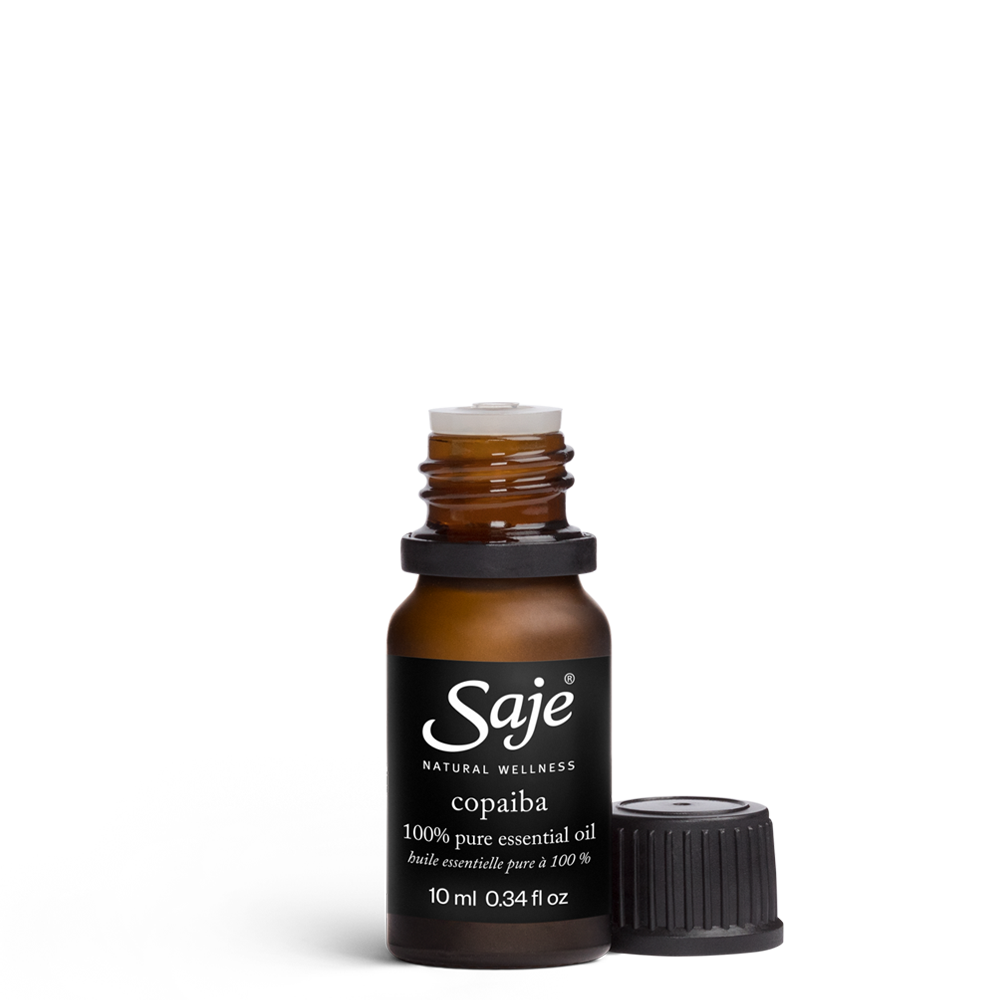This photograph features a small, high-end amber-colored bottle labeled "Saje Natural Wellness 100% Pure Essential Oil." The bottle, which holds 10 milliliters (0.34 fluid ounces) of essential oil, is topped with a pale white, short stopper cap designed to dispense drops sparingly. The cap is removed and positioned off to the right of the bottle on a pristine white background. The neck of the bottle has a slight spiral pattern that is accentuated by a black cylindrical separator, which leads to the main body of the bottle. The black label with white text on the front of the bottle details the product's name and the essential oil scent, Copaiba. Below the product name, the label also includes the size information in both milliliters and fluid ounces as well as the term "100% pure essential oil" in another language. Despite the lack of further descriptive instructions about the scent, the bottle itself reflects a sophisticated and likely premium product.